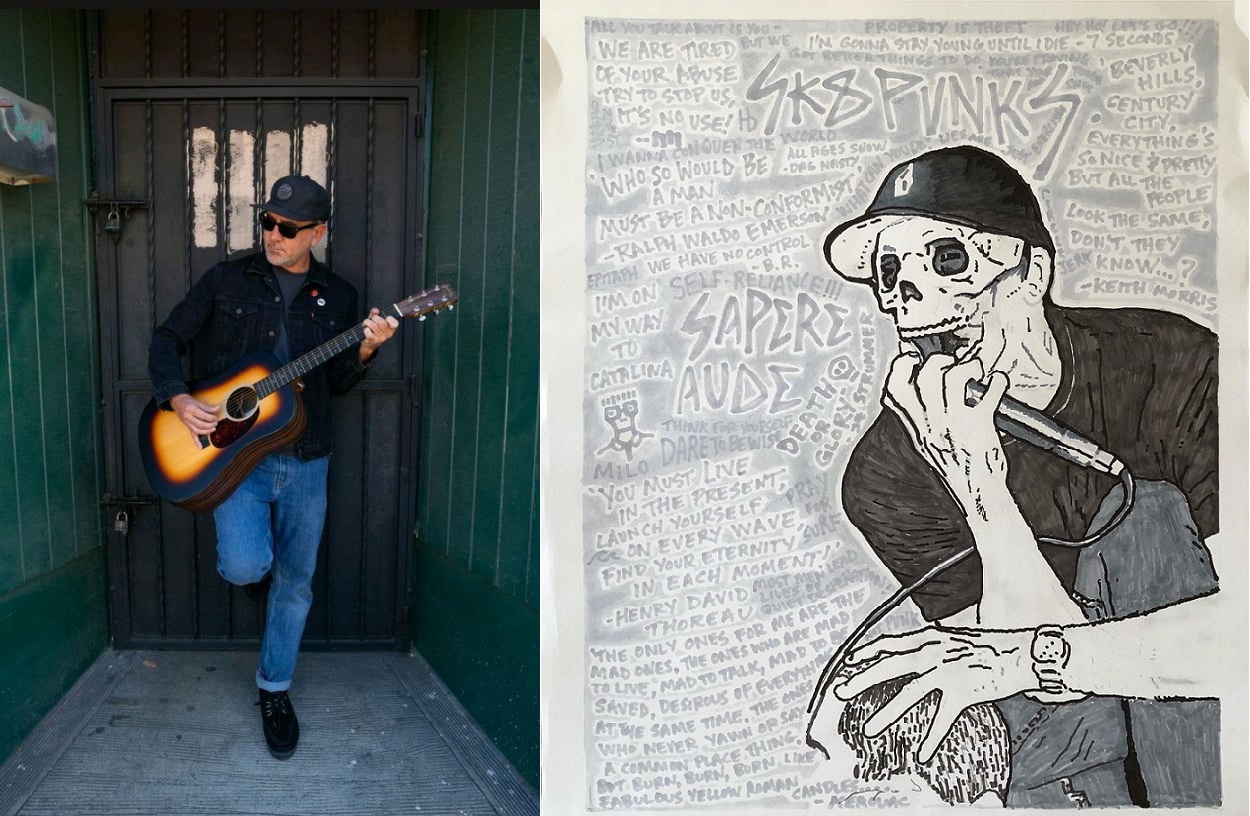This is a pair of side-by-side images, each in a rectangular format. The left image is a photograph of a man standing in a small entryway, characterized by green walls and a metal door with two padlocks and an obscured window segmented by pieces of wood, resembling four small windows that let light through. The man, dressed in a denim jacket, black jeans, black shoes, a baseball cap, and sunglasses, is playing an acoustic guitar. His upper hand is positioned on the chords while his lower hand strums. One of his legs is bent, with his knee forward and foot against the door behind him.

The right image is a pen-and-ink style illustration featuring a person with a skull mask, through which their eyes are visible. The figure is squatting, holding a microphone in one hand and resting the other hand on the top of another person's head. The background is filled with pale, gray text and graffiti-like quotes and writings. The heading "Skatepunks" prominently appears, linking the artistic motif to a subculture vibe. The drawn figure mirrors the man in the photograph, maintaining the same attire of a baseball cap and dark shirt, albeit with the skeletal facial twist suggesting a punk or rebellious theme.